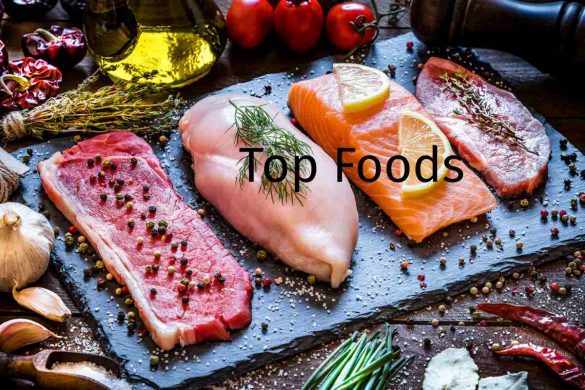This image appears to be a sophisticated advertisement for high-quality meats, meticulously arranged on a dark-colored, possibly slate, rectangular cutting board. The meats are placed diagonally, emphasizing a visually appealing layout. Starting from the left, there is a vibrant red steak adorned with black and white peppercorns. Adjacent to it lies a raw chicken piece garnished with green herbs, immediately followed by a fresh salmon fillet topped with two lemon slices. The display concludes with another cut of red meat, also sprinkled with green herbs.

Surrounding the central board are various cooking ingredients that add depth and context to the culinary scene. Black and red peppercorns are scattered across the presentation area, enhancing the gourmet feel. To the left, there are garlic cloves and onions, while red peppers and possibly tomatoes are positioned centrally at the top. An overturned pepper grinder and a jar that seems to contain olive oil sit to the side, along with chives placed at the bottom center. Additionally, dried garlic or pepper pods are noticeable in the foreground, along with a scoop possibly filled with salt.

The backdrop includes more scattered fruits, vegetables, and greenery, enriching the gastronomic setting. A bottle of wine or olive oil and various other colorful ingredients further embellish the scene. Overlaying the image in the center are the black letters spelling out "Top Foods," enhancing its appeal as an elegant and enticing food advertisement.